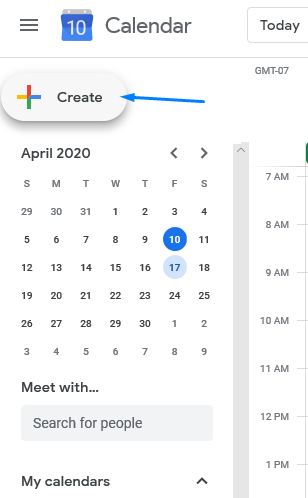The image showcases a screenshot of Google Calendar, specifically from April 2020. The interface features are as follows:

- **Top Left Corner:** The menu icon (represented by three horizontal lines) provides additional options when clicked.
- **Calendar Icon:** A blue box containing the number "10" next to the word "Calendar."
- **Today Button:** Located to the right of the calendar text.
- **Create Button:** Situated below the "Today" button, displaying a plus sign in Google's signature colors. A blue arrow is pointing at this button, indicating its significance.
- **Current View:** The month and year displayed are April 2020. The entire month is visible, with the 10th of April marked by a blue circle, highlighting it as a relevant date. Additionally, the 17th of April is highlighted in light blue, likely indicating it is the current date.

Below the date display:
- There's a search box labeled "Meet with" for finding people.
- The text "My calendars" appears beneath the search box.

**Right Side of the Screen:** Features a time slot grid from 7 AM to 1 PM for scheduling events.